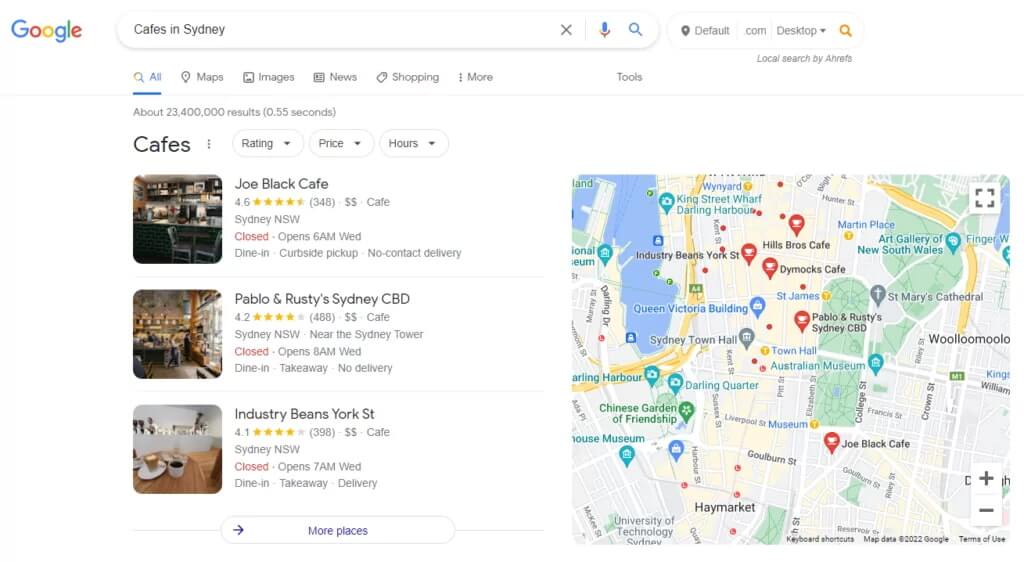Here's a cleaned-up and detailed caption for the described image:

---

This image is a screenshot of a Google search results page for cafes in Sydney, Australia. At the top of the page, there are various tabs such as 'All,' 'Maps,' 'Images,' 'News,' 'Shopping,' and 'More,' sitting just below the search bar. The search generated approximately 23,400 results in 0.55 seconds. Below these tabs, there are filtering options allowing users to sort cafes by rating, price, and hours of operation.

The first result is Joe Black Cafe, which boasts a rating of 4.6 stars based on 348 reviews. It is categorized as a moderately priced cafe located in Sydney, NSW. The cafe is currently closed but will open at 6 a.m. on Wednesday and offers dine-in, curbside pickup, and no-contact delivery options. The image associated with Joe Black Cafe shows a pair of chairs pushed against a countertop.

The second result is Pablo and Rusty's Sydney CBD, with a rating of 4.2 stars from 488 reviews. This cafe also falls into the moderate price range and is located near the Sydney Tower in Sydney, NSW. It is similarly closed, reopening at 8 a.m. on Wednesday, with dine-in and takeaway services available, but no delivery. The image shows people walking inside the cafe.

The third result is Industry Beans on York Street, holding a 4.1-star rating from 398 reviews. Like the previous cafes, it is categorized within a moderate price range in Sydney, NSW. It is currently closed and will reopen at 7 a.m. on Wednesday, offering dine-in, takeaway, and delivery services. The accompanying image displays multiple cups of coffee or tea arranged on a table.

On the right side of the screenshot, there is a map highlighting the locations of various cafes in Sydney. The map includes notable landmarks such as the Australian Museum and the Town Hall, helping to show the geographical relation of the cafes in relation to these landmarks. Specific cafes like Domics Cafe and St. James are also marked on the map.

---

This detailed description provides a comprehensive overview of the search results and includes visual details of both the listings and map presented in the image.